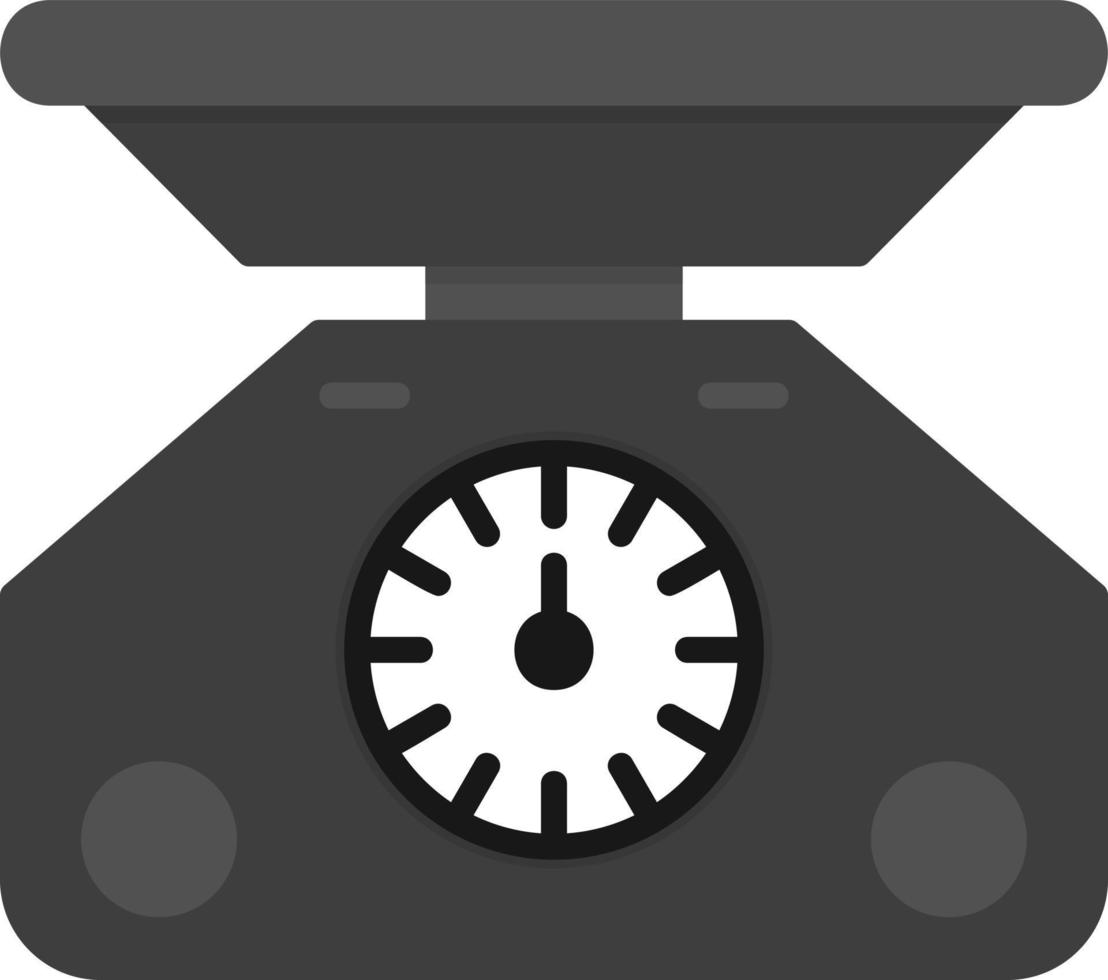This image features a detailed, stylized drawing of a large scale, occupying the entire frame against a white background. The scale is depicted primarily in gray, black, and white tones. At its base, there is a trapezoidal structure with a central, round white dial, reminiscent of a clock face, but without numbers. Instead, black markings encircle the dial, signifying different weights, with a stationary black arm pointing at zero, indicating the scale is empty. Flanking this dial are two gray round knobs or circles positioned at the bottom left and right corners of the base, possibly serving as adjustment controls. Above the dial, two gray lines are present, though their function is unclear. The weighing platform, which resembles a rectangular or upside-down trapezoidal tray, is positioned at the top. This tray is black with a hint of gray at the upper edge, designed to hold items, and is reminiscent of an old-fashioned meat scale. The overall design is simple yet detailed, capturing the essence of a traditional weighing device.